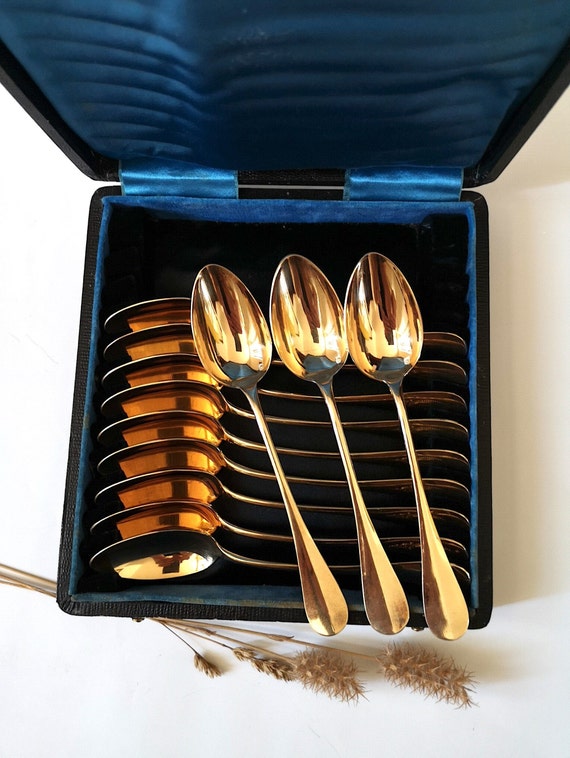The image depicts a collection of gold-colored spoons arranged in a blue velvet-lined box, which is partially open. There are a total of twelve spoons, with nine spoons neatly positioned side by side with their bowls facing to the left, and three additional spoons laid horizontally atop the others with their bowls facing upward. The spoons, which are reflective and well-polished, appear to be used, as indicated by subtle scratches on their handles, suggesting they are not brand new. The box, casting a shadow to the right, rests on a white surface. Below the box, beige-colored wheat grains with fluffy stalks add a natural element to the composition. This professional image emphasizes the uniqueness and special status of the spoons, highlighted by their organized presentation in a luxurious blue container.